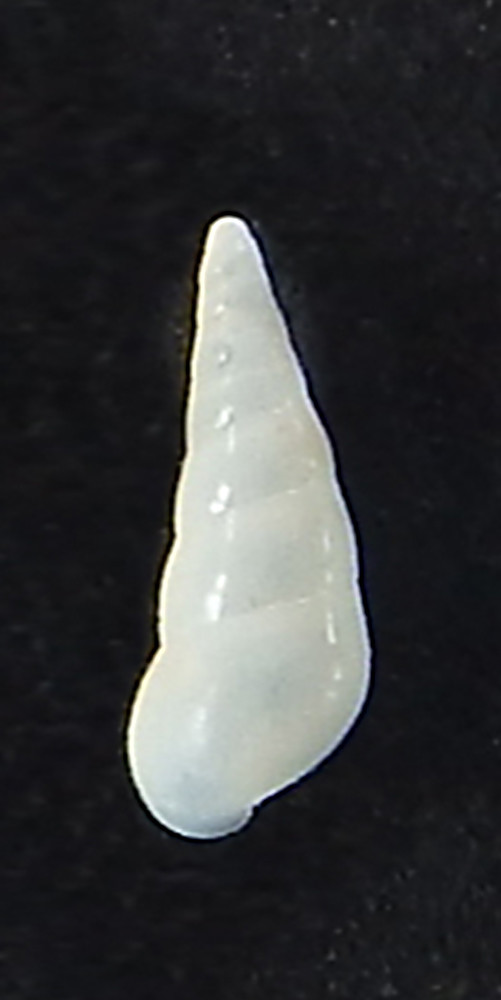The image shows a striking white object, likely a polished seashell, set against a completely black background. The shell, which has a smooth, translucent appearance and a shiny surface, somewhat resembles a delicately sculpted horn or an upside-down ice cream cone. It is shaped with a pointed tip at the top, gradually widening towards the bottom, embodying elegant swirls akin to those found on seashells or snail shells. The photoshoot highlights the shell's pristine, crisp whiteness and a slight texture against the black backdrop, accentuating its luminous presence. The image itself is taller than it is wide, emphasizing the vertical elegance of the seashell, which stands prominently as the sole subject of the photograph.